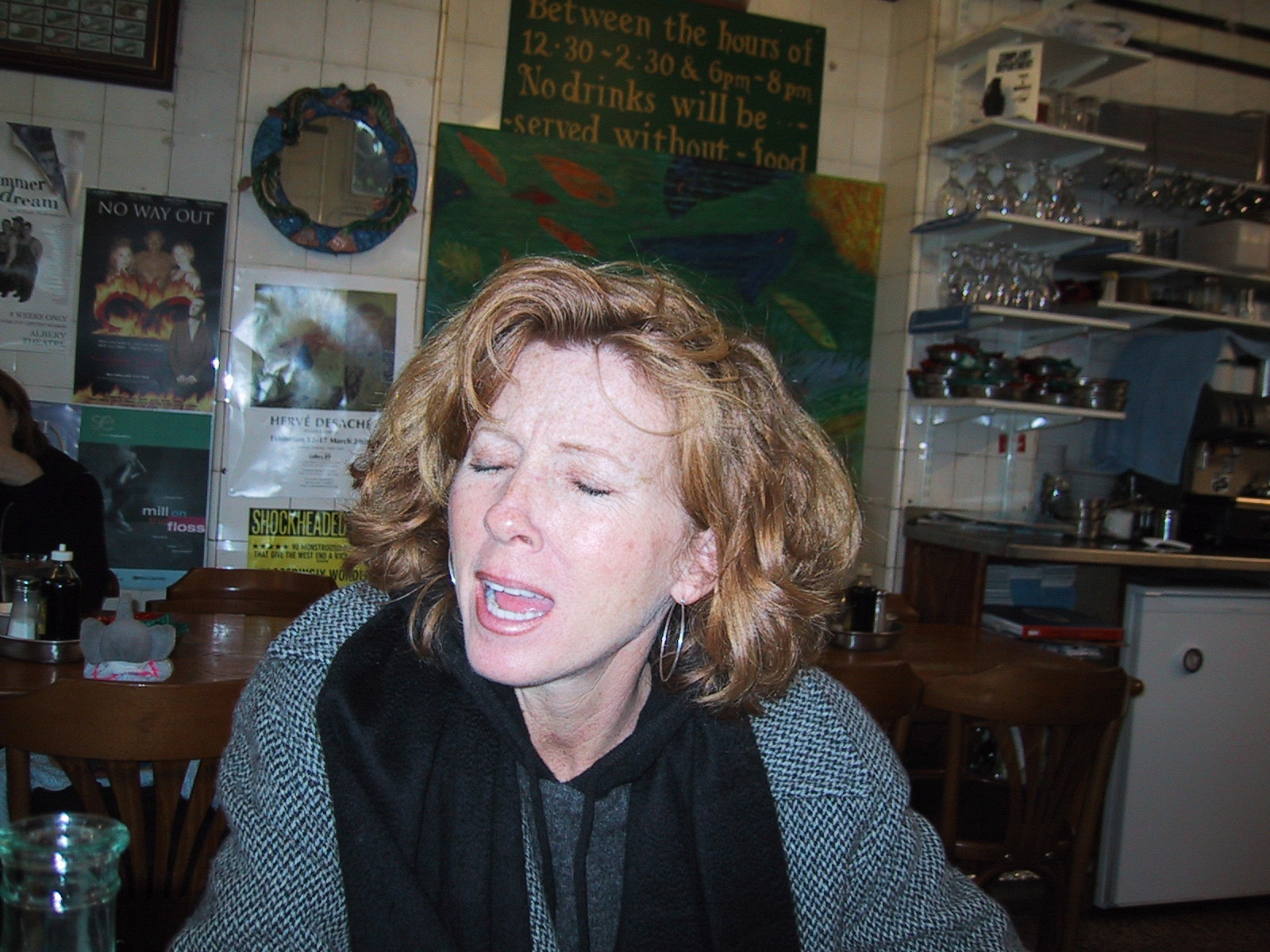The photograph features a fair-skinned, white woman who appears to be in her middle age. She has auburn to strawberry blonde hair parted down the middle, and she is adorned with large silver hoop earrings. Her eyes are closed and her mouth is open, indicating she might be singing. She is dressed in a gray sweatshirt layered with a gray herringbone or tweed coat and a black scarf. Her lips have a subtle gloss. The background suggests she is in a kitchen or a restaurant, given the shelves filled with drinking glasses and various objects on the counter. Additionally, there are multiple posters or printouts and a clock on the wall behind her. A notable detail includes a green sign with yellow text, which partially reads, "No drinks will be served without food between the hours of 12:30 through 2:30 and 6 p.m. through 8 p.m." The scene also shows tables with chairs and condiments, further hinting at a restaurant setting.